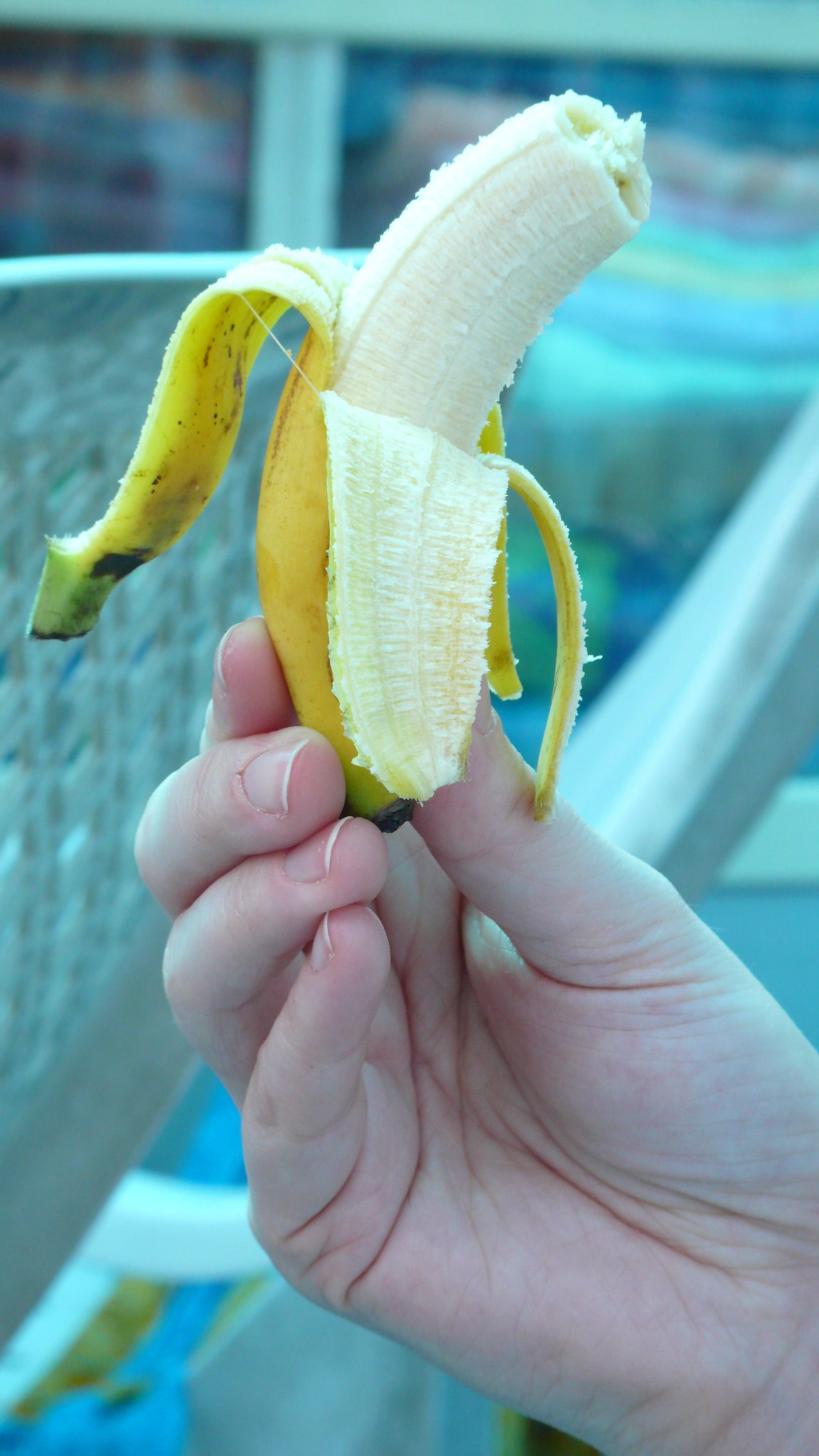The image features a well-manicured woman's hand holding a small, peeled banana. She grips the banana delicately between her thumb, forefinger, and middle finger of her right hand. A bite has been taken from the banana, revealing the white fruit inside. The banana appears to be a variety smaller than the typical supermarket banana, possibly a type of plantain. In the background, there is a metallic railing alongside a white window frame. The glass in the window offers a hazy, blurred view of the outdoors. To the left of the frame, a woven, lattice-style material—likely from an outdoor patio chair—adds texture to the scene.